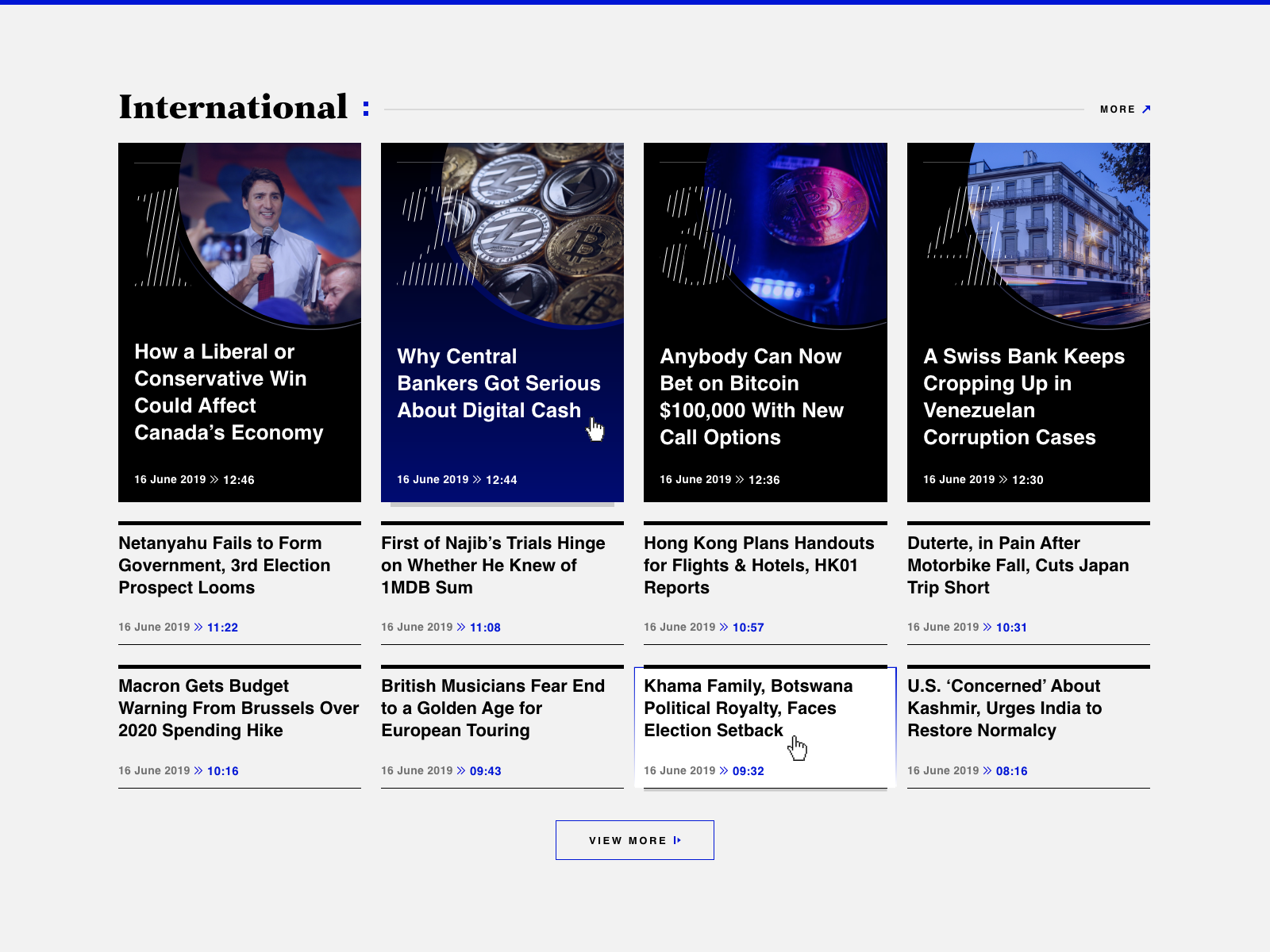**Detailed Image Caption:**

The web page features an international news section beginning with a heading that reads "International" but does not include a web link. On the left side of the web page's layout, the right side has an option labeled "Click for more." 

The page prominently displays four images with news headlines and timestamps:

1. **Image 1**: A man is seen standing and speaking into a microphone, possibly presenting or engaged in a discussion. The accompanying heading reads, "How Liberal or Conservative Win Could Affect Canada's Economy." The image is timestamped June 16, 2019, at 12:45.
   
2. **Image 2**: Depicts various bitcoins and other forms of digital currency. The heading states, "Why Central Bankers Got Serious About Digital Cash," with a timestamp of June 16, 2019, at 12:44.

3. **Image 3**: Shows the number "30" alongside a coin, hinting at financial or betting themes. The headline here is, "Anybody Can Now Bet on Bitcoin $100,000 with New Call Options," timestamped June 16, 2019, at 12:36.

4. **Image 4**: Features a building resembling a hotel with the headline, "Swiss Bank Keeps Cropping Up in Venezuelan Corruption Cases," timestamped June 16, 2019, at 12:30.

Below these images, the web page lists various clickable section headings with news titles, each related to international affairs and all dated June 16, 2019. The headings include:

1. "Netanyahu Fails to Form Government; Third Election Prospect Looms."
2. "First Najib's Trials Hinge on Whether He Knew of 1MDB."
3. "Hong Kong Plans Handouts for Flights and Hotels, HKO1 Reports."
4. "Duterte in Pain After Motorbike Falls; Cuts Japan Trip Short."
5. "Macron Gets Budget Warning from Brussels Over 2020 Spending Hike."
6. "British Musicians Fear End to a Golden Age for European Touring."
7. "Khama Family, Botswana Political Royalty, Faces Election Setback."
8. "U.S. Concerned About Kashmir, Urges India to Restore Normalcy."

Each of these headings provides a brief insight into significant political, economic, and social issues from around the world.